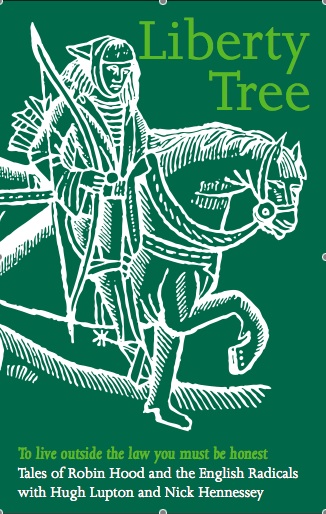The image appears to be a book cover with a medium-tone green background. At the top right corner, the title "Liberty Tree" is displayed in light lime green text. Dominating the cover is a large, detailed white line illustration. This illustration, which occupies about 90% of the cover, depicts a medieval scene featuring a man in old-timey clothes riding a horse, holding a bow with arrows in a quiver on his back. The scene evokes a sense of historic and legendary storytelling. Below this illustration, in lime green text, is the quote "To live outside the law, you must be honest," and beneath that, in white text, it says "Tales of Robin Hood and the English Radicals with Hugh Lupton and Nick Hennessy." The edges and corners of the image have small gray circles, reminiscent of cropping marks seen in photo editing software like Photoshop.